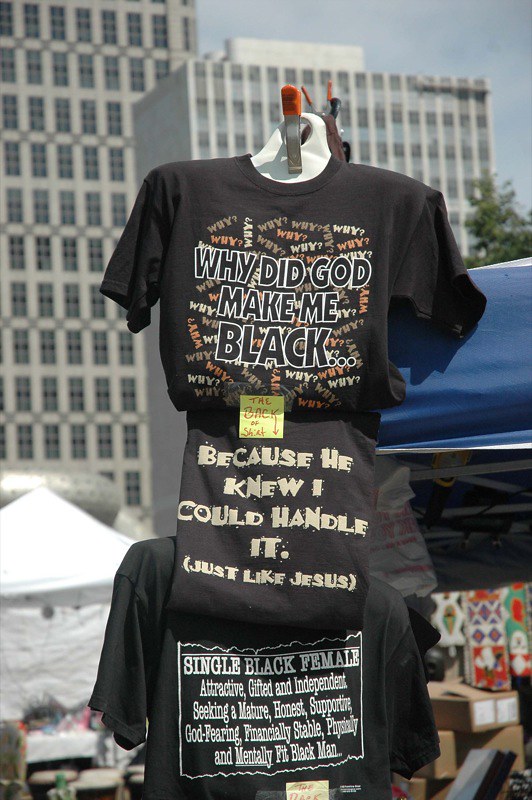The image is taken outdoors and portrays a scene likely set in a bustling flea market or vendor fair, with various small businesses and vendors offering products. At the center, two black t-shirts are displayed prominently. The top t-shirt bears bold white text reading, "Why did God make me black?" with numerous colorful "why" questions scattered in the background. Affixed to this shirt is a sticky note pointing downwards, indicating, "The back of the shirt." Below it, presumably showcased as the backside, is a t-shirt with the text, "Because He knew I could handle it," followed by, "just like Jesus" in brackets. Adjacent to these shirts, another one features a personal ad with white text on a black background: "Single Black female, attractive, gifted, and independent, seeking a mature, honest, supportive, God-fearing, financially stable, physically and mentally fit Black man," with "mentally" underlined. Surrounding the display are tents, boxes, and other items suggesting a market setting, while tall skyscrapers loom in the distant background, situating the scene within a lively urban environment.